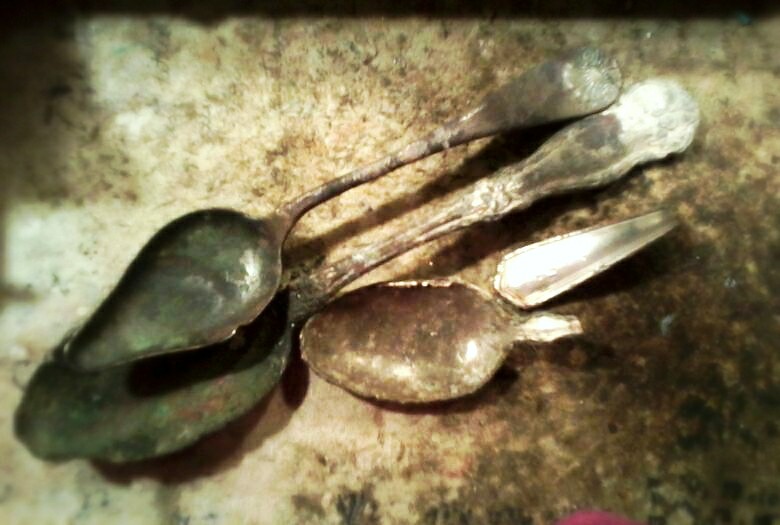This monochrome photograph captures a collection of three antique spoons, each exhibiting signs of extensive rust and age, creating a striking visual against a moldy, textured background. The base of the image, mottled with dark gray and brown hues, transitions to a softer, aged paper-like appearance towards the center. Diagonally arranged from the bottom left to top right, two intact spoons showcase dull pea soup green and black bowls, slashed with faded silver handles adorned with faint, intricate designs. Below and between these spoons lies the bowl of a fragmented spoon, its handle placed separately but aligned, both pieces heavily tarnished. The spoons, possibly unearthed relics, evoke an underwater shipwreck or archaeological dig, their surfaces calcified and encrusted with dirt, depicting a grim testament to the ravages of time.